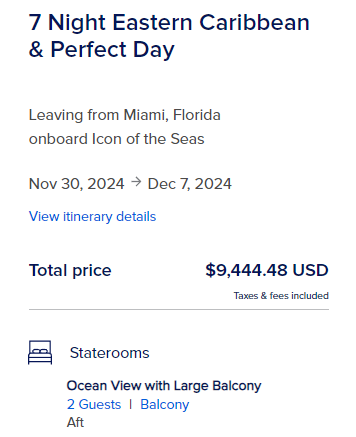The image displays a snapshot of a cruise ticket for a luxurious journey titled "Seven Night Eastern Caribbean and Perfect Day." This title is prominently placed at the top in bold, eye-catching text. Directly beneath this, there is a smaller, slightly less bolded line of text reading, "Leaving from Miami, Florida, Onboard Icon of the Seas." The cruise dates are clearly specified, running from November 30th, 2024, to December 7th, 2024, with an arrow indicating the duration. 

Below the dates, there's a clickable hyperlink that says, "View itinerary details." At the bottom portion of the image, the total price of the cruise is displayed prominently: $9,444.48 USD. Below the price, in very small text, it is noted that this amount includes all taxes and fees. A thick horizontal line separates this section from the next part of the screenshot. 

The lower section features an icon of a bed accompanied by the text, "State Rooms," indicating that the accommodation includes an "Ocean View Large Balcony" room.